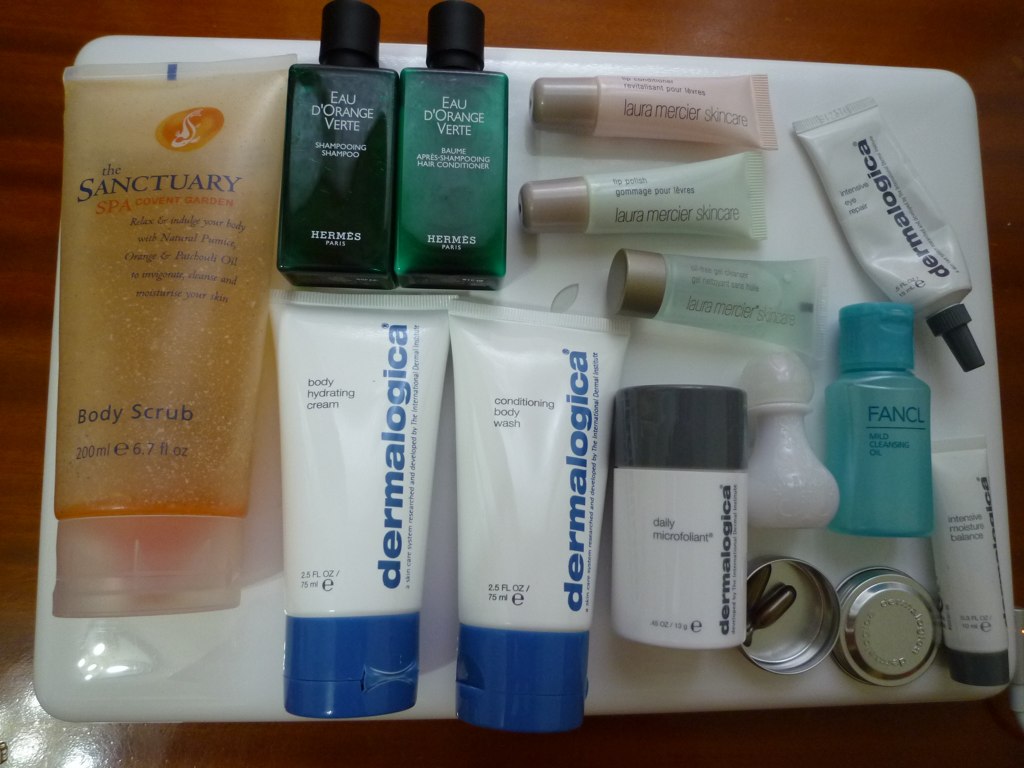This image features a meticulously arranged make-up tray housing a collection of 13 distinct items set against a wooden background. On the left, a body scrub by The Sanctuary takes the spotlight in a translucent bottle, showcasing its vibrant orange contents. Adjacent to this, two green bottles of Eau d'Orange Verte shampoo and conditioner from Hermès, Paris, occupy the top center.

Directly below, two elegant bottles of Dermalogica's body hydrating cream and conditioning body wash stand side by side. Nestled beside them, a compact daily microfoliant from Dermalogica adds to the skincare collection. 

Towards the middle right, three lip treatments by Laura Mercier Skin Care, in pink, green, and translucent aqua shades, highlight varied options for lip care. At the top right corner, another Dermalogica bottle stands prominently, enhancing the brand's representation on the tray.

Down at the bottom, an unmissable small pillbox is placed thoughtfully, accompanied by a petite pink bottle just above it. Nearby, a small bottle from Fancel introduces another brand into the mix, while a final small Dermalogica tube rests on the far right.

Set on a pristine white tray, the assortment features a diverse palette including orange, green, white with blue lettering and caps, gray, and the mentioned aquamarine, creating a visually appealing and organized presentation.